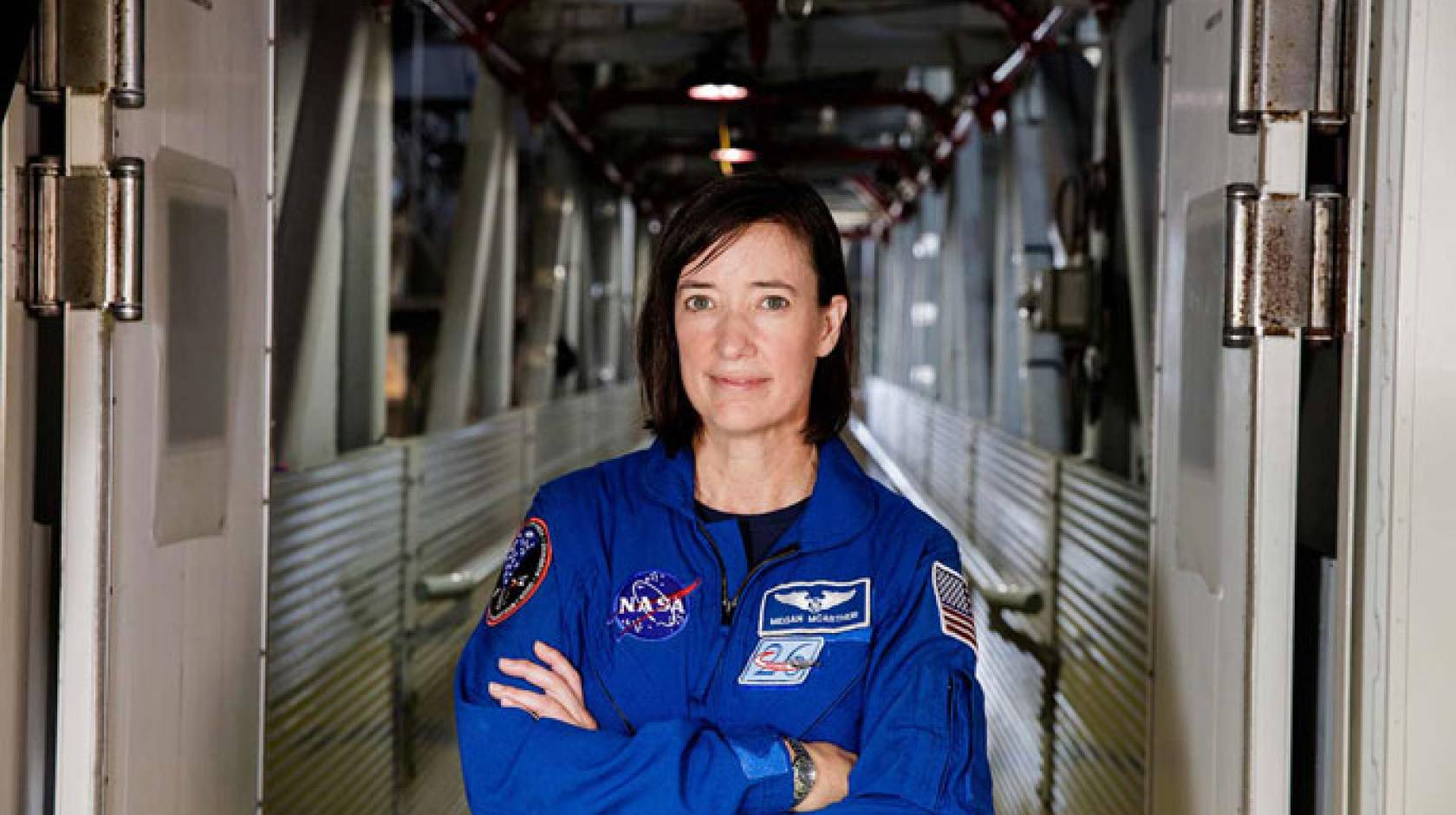This photograph captures a close-up of a female astronaut standing in a narrow, metallic corridor that appears to be part of a gantry or an access point to a space capsule. The astronaut has shoulder-length, dark hair and big, bluish-green eyes, and she is smiling slightly at the camera. She wears a blue NASA jumpsuit, which features multiple patches and emblems. On her left breast is the customary NASA logo, while her right shoulder bears an American flag patch. In addition, there’s a name badge that is hard to read, but possibly says "Megan McCarter." Below the name badge is a patch displaying the number "26" with a red and orange swoosh through it. Another notable patch on her left arm has a red outline, a black interior, and a blue triangle in the center, with white writing near the red border. The jumpsuit has a central zipper revealing a dark blue t-shirt underneath. She stands with her arms crossed, one arm resting under her right arm and the other on top of her left arm. The surrounding corridor has shoulder-high corrugated steel walls, railings, and triangular girders, suggesting structural support consistent with access tunnels in a space facility. The scene is illuminated by overhead lights, highlighting the metal textures and creating a focused atmosphere as she stands in the open doorway with metal doors hinged on either side.